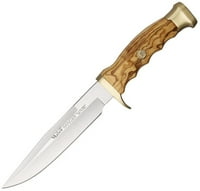In this image, set against a completely white background, there is a single object positioned diagonally from the top right to the bottom left. It is a medium-length knife, likely a steak knife, with a blade made of smooth, silver metal. The blade bears the somewhat challenging-to-read text "Mucklay Ranger," presumably indicating the brand name. The handle is made of a light brown wood with darker brown squiggly lines, and it features a small gold metal piece at its tip. Additionally, there is a single metal circle in the middle of the handle whose details are unclear. This image is reminiscent of product photos typically seen on websites selling knives or sporting goods, showcasing the knife's details and quality.